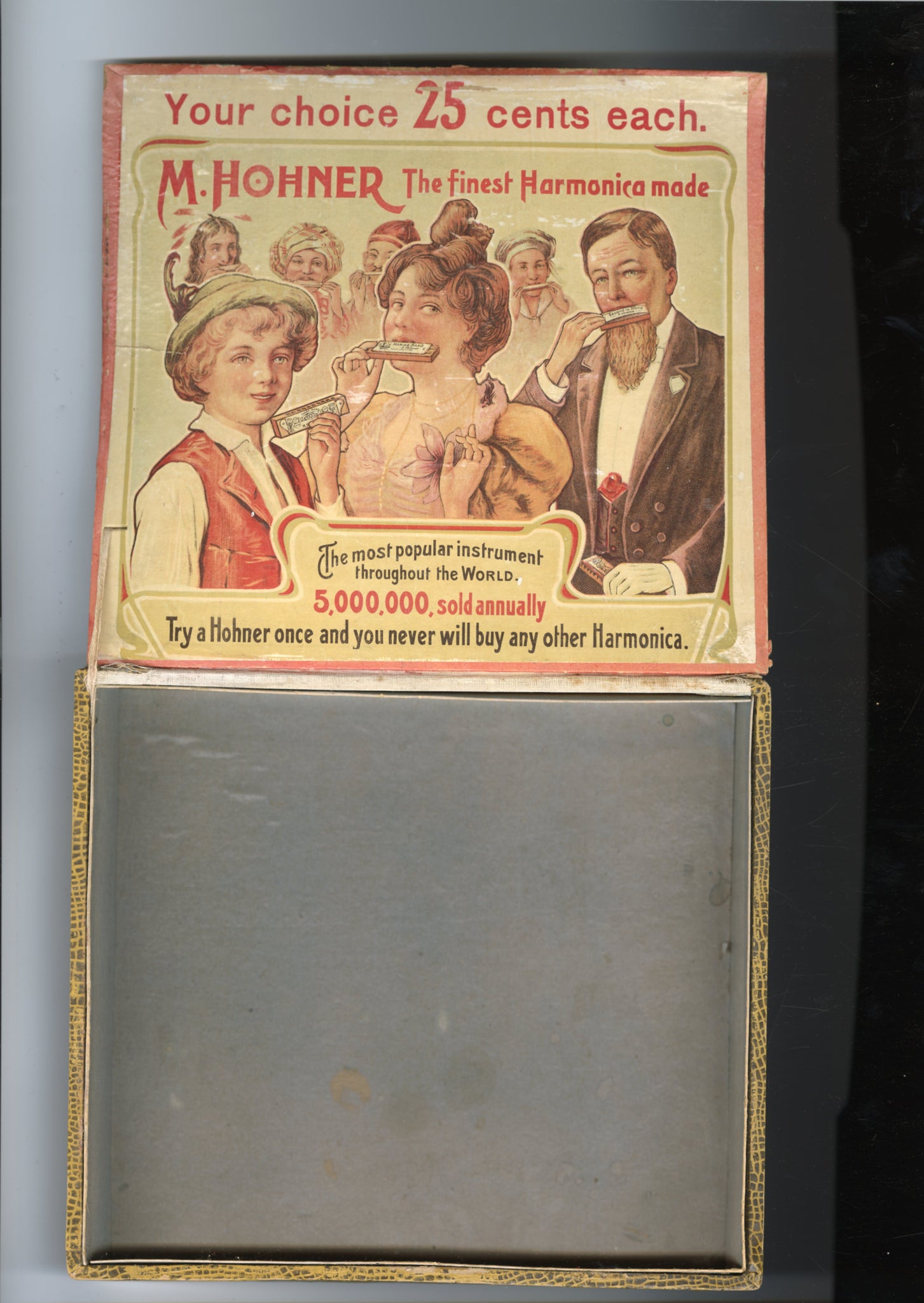This is an old-fashioned advertisement for M. Hohner harmonicas, showcasing a nostalgic atmosphere possibly from the late 1800s or early 1900s. The ad features seven people, including men, women, and a boy, dressed in vintage attire. Some hold harmonicas to their mouths, poised to play, while others simply display them. The text at the top of the ad, in striking red capital letters, reads, “Your choice, 25 cents each, M. Hohner” followed by, “The finest harmonica made.” Additional text emphasizes its global popularity: “The most popular instrument throughout the world, five million sold annually. Try a Hohner once, and you'll never buy any other harmonica.” The entire ad has a faded, yellowish hue, with alternating black and red text, and a red border surrounding the imagery. Beneath the advertisement is a plain, chalkboard-like box that may be the packaging for the harmonica, all set against a black curtain and gray background.